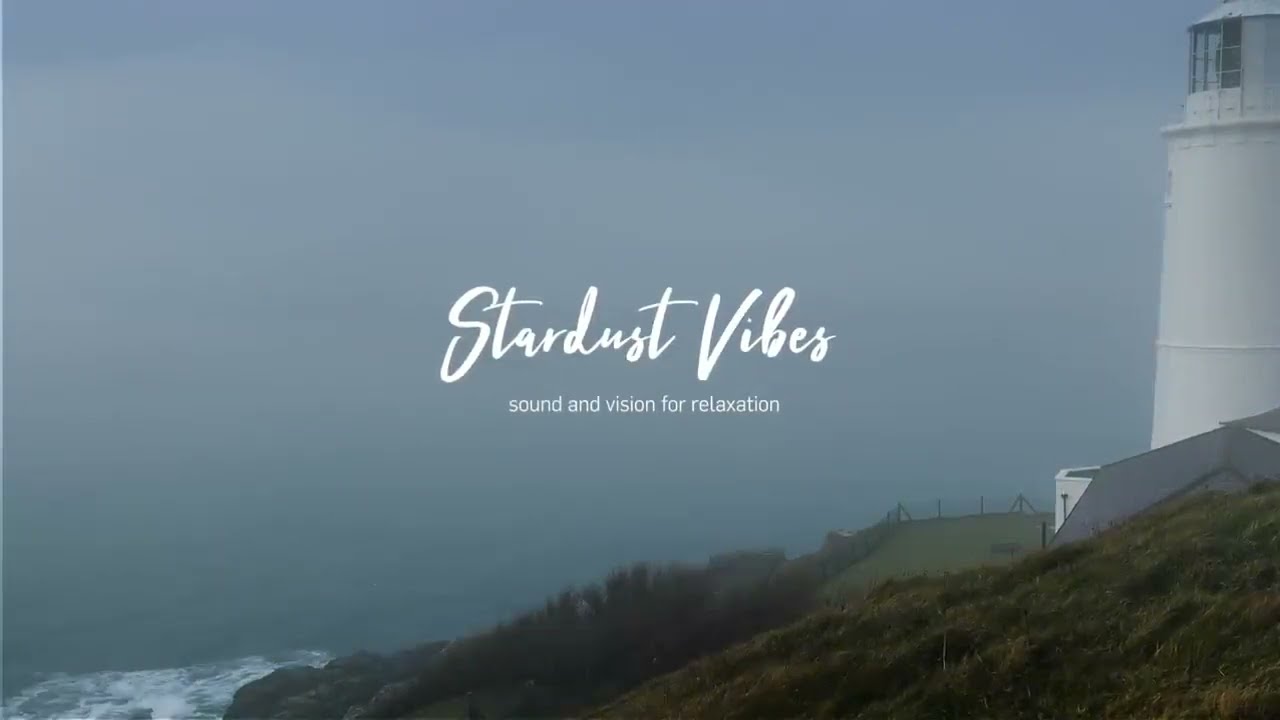The image features a white lighthouse positioned on the right side, perched high on a cliff beside a green, mountainous hillside abundant with grass, vegetation, and trees. The left and most of the image is dominated by the sea and a cloudy sky, creating a nearly seamless blend at the horizon. Noticeable are the white-capped waves crashing close to the shore. Overlaying this serene landscape, in the center of the image, there is cursive white text reading “Stardust Vibes,” followed by a smaller line underneath that says, “Sound and Vision for Relaxation.” The scene exudes a calming atmosphere with a color palette featuring whites, blues, greens, browns, and grays, indicative of an overcast day, and there are no people visible in the frame.